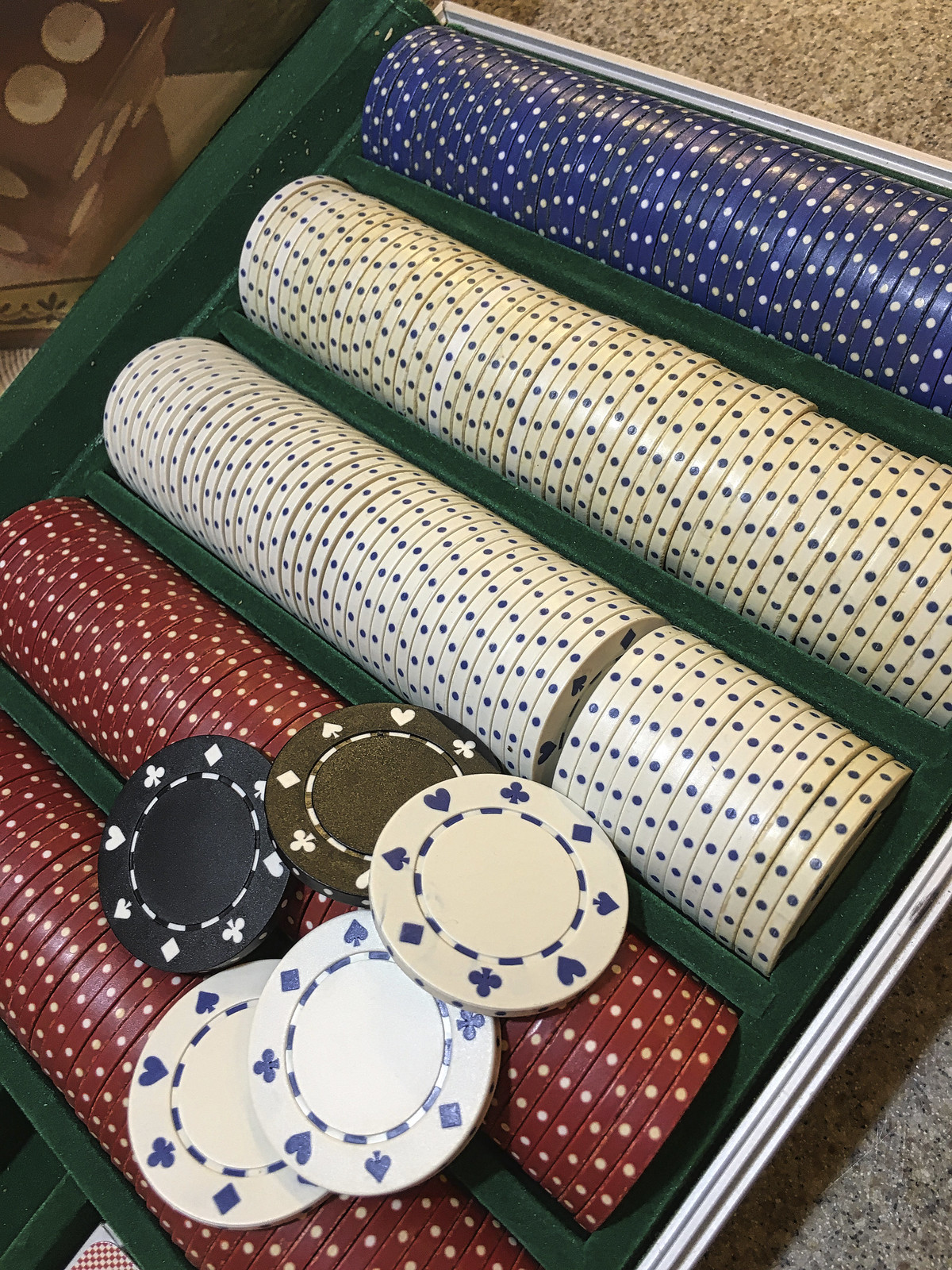A detailed close-up image of a collection of poker chips, neatly organized in a green velvet tray. The chips come in various colors: white with blue hearts, spades, clubs, and diamonds, bordered with white polka dots; red with red and white polka dots, decorated with matching red suits around the edges; solid black, blue, and brown chips are also visible, each meticulously stacked. The tray includes a portion of a deck of cards, hinting at a classic gambling setup. The entire arrangement rests on a gray surface, potentially a countertop or piece of cloth, accented by a metallic rim around the tray, enhancing the luxurious feel of the setting.